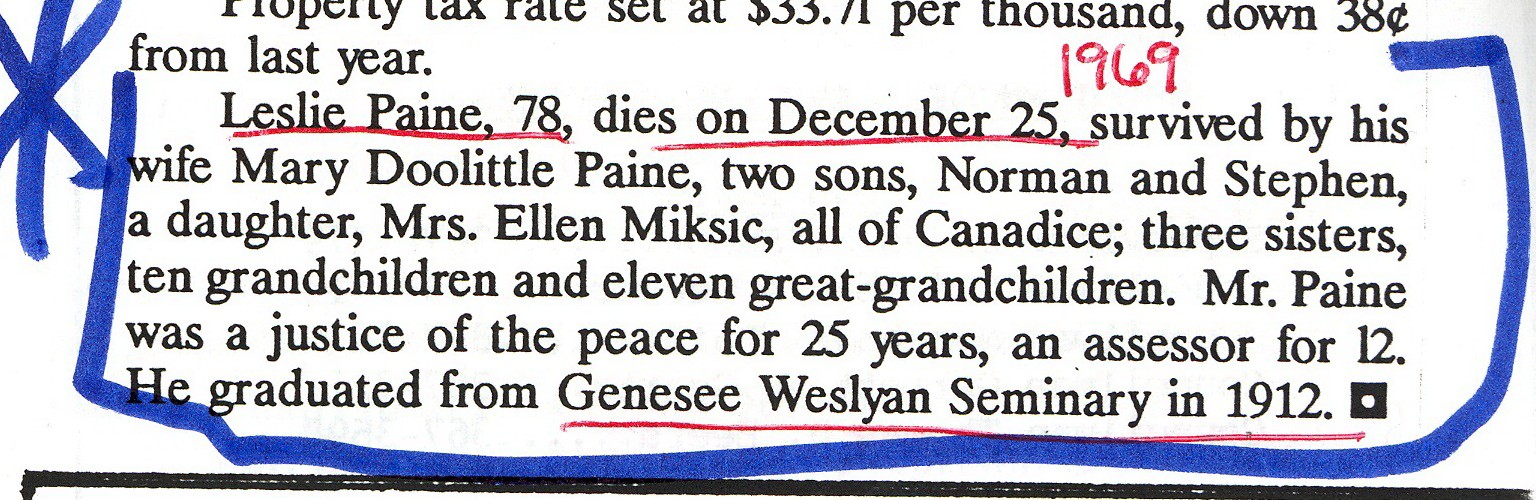The image appears to be a clipping from a newspaper article, extensively marked with various colored inks. A paragraph bordered by thick blue marker, with a blue star on the left side, details the obituary of Leslie Payne, 78, who passed away on December 25, 1969. The key details "Leslie Payne, 78," "dies on December 25th," and "1969" are underlined in red ink. Payne is survived by his wife, Mary Doolittle Payne, two sons, Norman and Stephen, and a daughter, Mrs. Ellen Miksic, all of Canadis. He also leaves behind three sisters, ten grandchildren, and eleven great-grandchildren. Notably, Leslie Payne served as a Justice of the Peace for 25 years and as an Assessor for 12 years. He was an alumnus of the Genesee Wesleyan Seminary, graduating in 1912—a fact also underlined in red ink. The paragraph begins with some context cut off, mentioning a property tax rate of $33.71 per thousand, slightly reduced by 38 cents from the previous year.